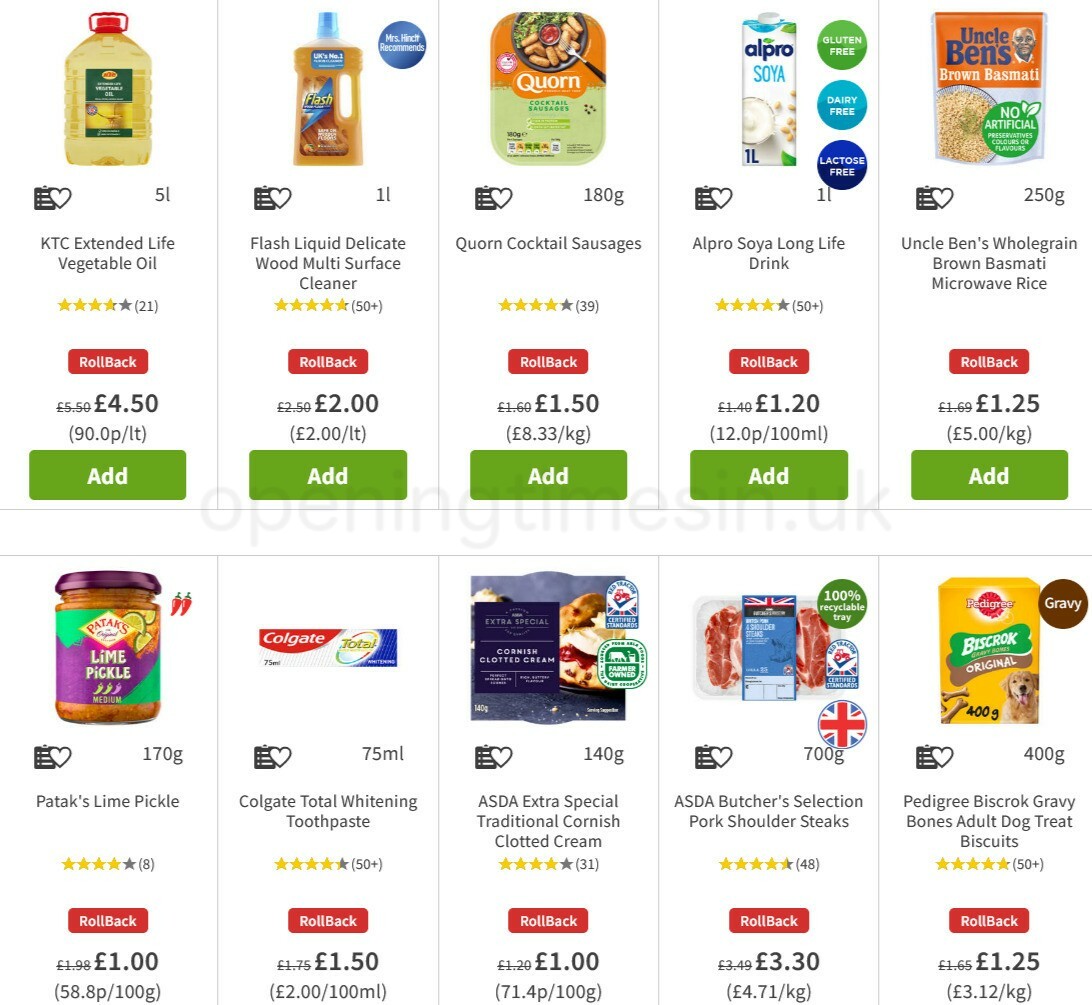In this image from a section of a store, we observe a white background with two rows of five food and household items each, totaling ten items. On the top row, starting from the left, we see a bottle of KTC Extended Life Vegetable Oil, followed by a Multi-Surface Cleaner for wood. Next, there are Cocktail Sausages, a Long-Life Soya Drink, and a packet of Uncle Ben's Brown Basmati Rice. Moving to the bottom row, from the left, there is a jar of Patak's Lime Pickle, a tube of Colgate Total Whitening Toothpaste, a container of ASDA Extra Special Traditional Cornish Clotted Cream, a pack of ASDA Butcher's Selection Pork Shoulder Steaks, and finally, a box of Pedigree Biscrok Gravy Bones dog treats. Below all these items, there is a rollback tab indicating the discounted prices.